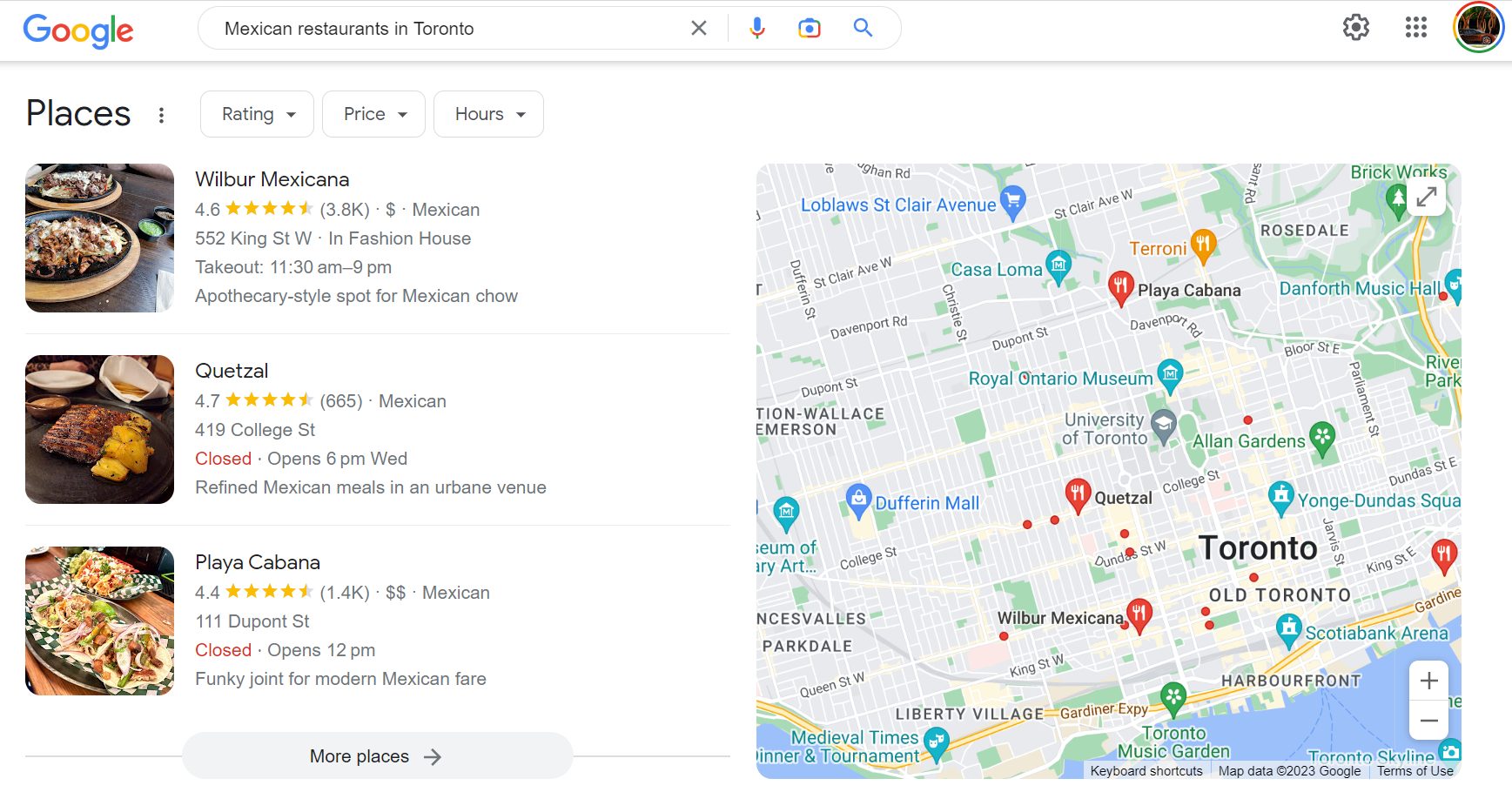The image is a screenshot of a Google Maps search page for Mexican restaurants in Toronto. At the top of the image is a horizontal bar featuring the multicolored Google logo on the left. Adjacent to the logo is a search bar filled with the query "Mexican restaurants in Toronto." To the right of the search bar are a microphone icon for voice search and a magnifying glass icon for text search. On the far right of the top bar, there are icons for settings (depicted as a small cogwheel) and the user's Google profile image.

The central section of the screen is divided into two main parts. On the left, the word "Places" is displayed in bold black text. Below it, three restaurants appear as search results: Wilbur Mexicana, Quetzal, and Playa Cabana. Each restaurant listing includes details such as operating hours, location, price range, and links to Google reviews.

On the right side of the screen is an overlaid map of Toronto, Canada. Red dots mark the locations of the aforementioned restaurants, providing a visual representation of where they are situated within the city. Additional red dots indicate more Mexican restaurants in the area. In the bottom left corner of the image, a "More Places" option allows for an expanded search.